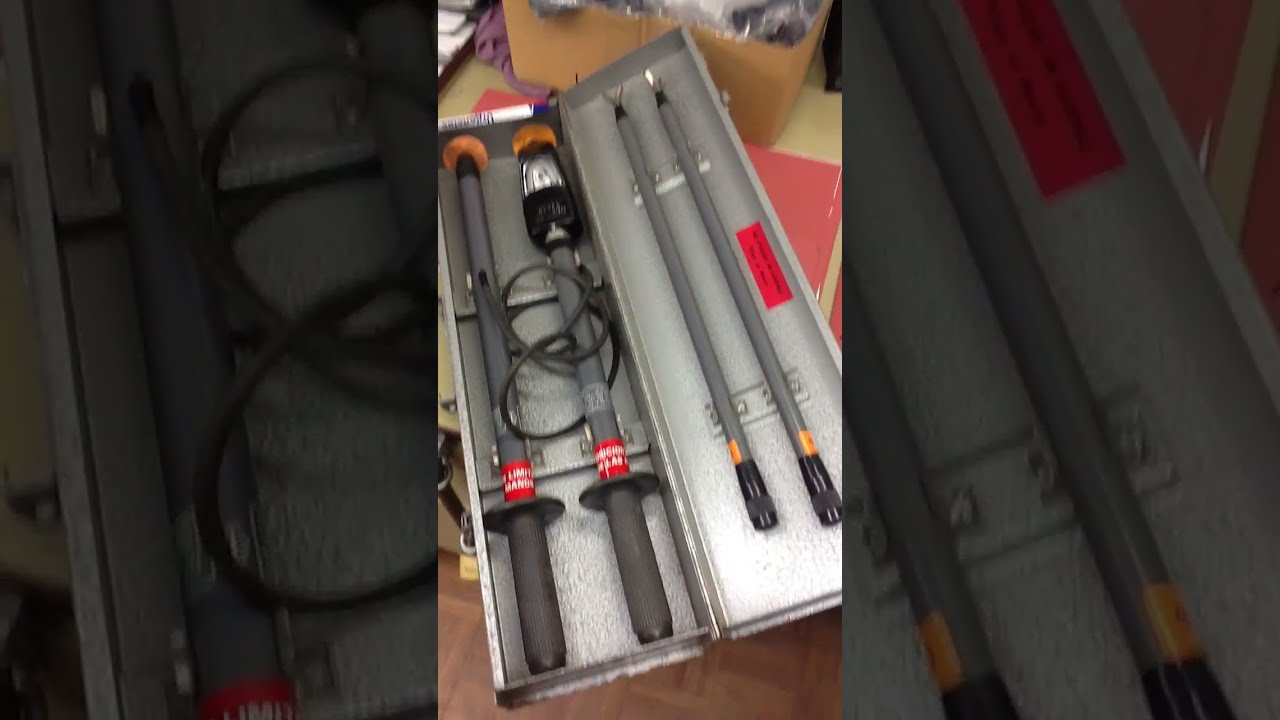The image depicts an open steel container housing several tools that resemble police batons or sword-like implements. Each tool features black rubber handles with circular guards resembling sword hilts. Above the handles are gray poles with orange tips on some, and the left pole is uniquely marked with red tape just above the handle. Some tools have yellowish or metallic tips, while others have two-pronged, sharp metal tips. Additionally, one of the gray poles on the right side includes a black meter with a white gauge, and black tubing is wrapped around it. There is also a black device with a groove cut out, attached to one of the tools, forming an upside-down U shape. The inside of the container also appears to have some Spanish text, though it is partially obscured and blurry. The box itself contains black framing components and an additional part which seems like a replacement or an attachment, stored towards the top.